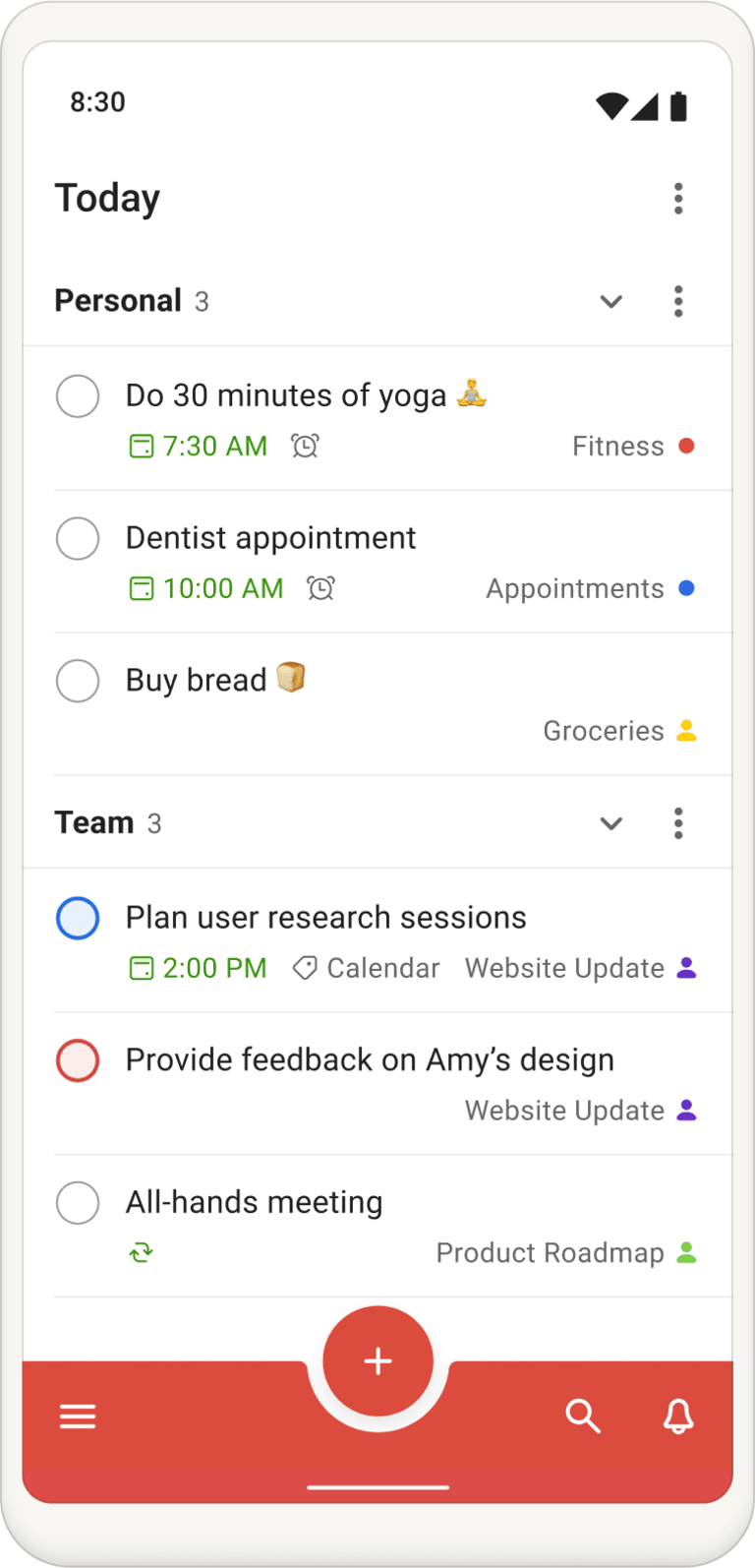In this detailed image, a cell phone screen is displaying an agenda app with a clean, white background. The status bar at the top of the screen shows the current time as 8:30, with Wi-Fi, cellular signal, and battery indicators on the top right. Below, the main interface of the app features a chronological list of tasks, each associated with a specific time when applicable. The tasks include "Do 30 minutes of yoga" at 7:30 a.m., "Dentist appointment" at 10 a.m., and "Buy bread" with no specified time. Each task is preceded by a circle on the left, acting as a checkbox for completion.

Further down, the app appears to separate personal tasks from team-related tasks, the latter of which include "Plan user research assessments," "Provide feedback on Amy's design," and "All hands meeting." 

The bottom right-hand corner of the screen houses two functional icons: a magnifying glass for searching and a bell for notifications. The design is minimalistic, focusing on ease of use and clarity in managing daily tasks.